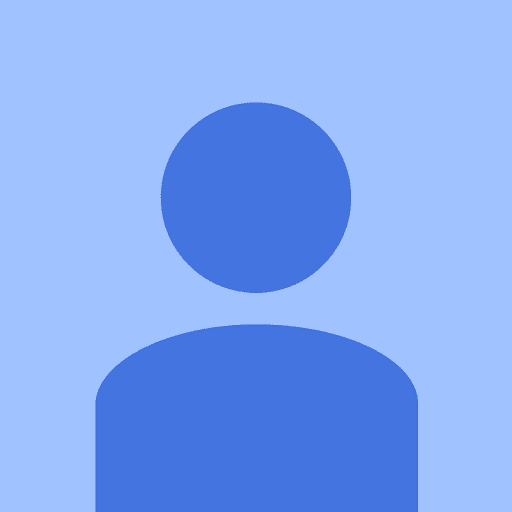The image captures a dynamic scene with a young boy energetically playing a large mustard yellow, or bronze-gold, drum set. Wearing an all-black outfit with a hoodie, the young drummer is seated on a classic round metal stool, and his drumsticks are raised mid-air, indicating vigorous action. The drum set, featuring five drums and three cymbals, dominates the foreground. The lighting creates a foggy effect with a black light shining down. His shadow is cast on the wall behind him, which appears to be a tan-colored or white sheet backdrop. The stage has a pinkish or red carpet. To the right in the background, two men are visible; one plays a guitar, and the other, possibly on a piano or keyboard, is partly cut off with his back facing the camera. Adjacent to them, a fan sits in the corner, adding to the casual atmosphere of what might be a concert or event. The overall scene captures the intensity and motion of the drummer with blurred hands and drumsticks, reinforcing the image's dynamic energy.